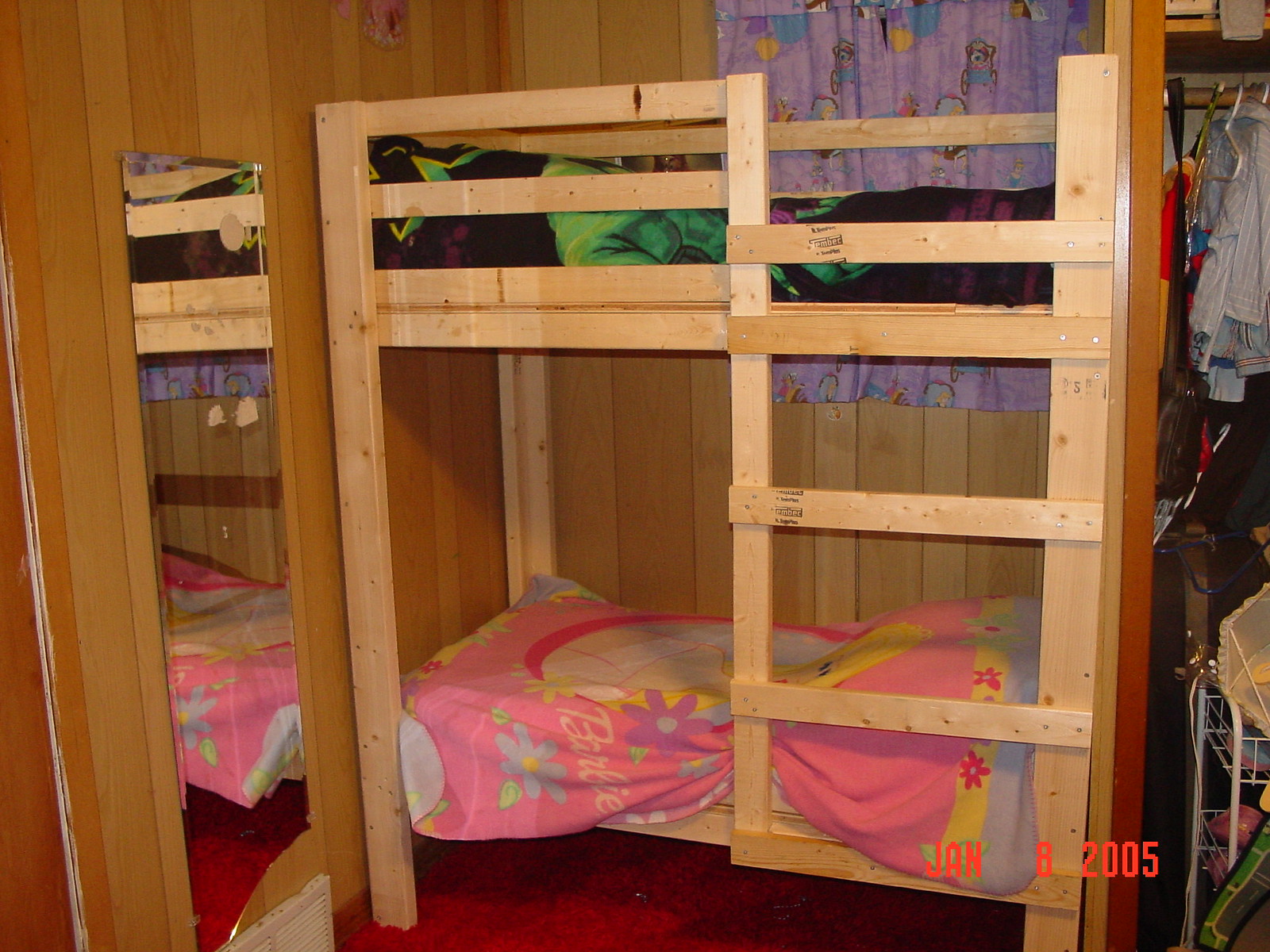This photograph, dated January 8, 2005, captures a cozy, makeshift children's bunk bed nestled against a light-colored wood-paneled wall. The bunk bed is crafted from light brown plywood, and features two short mattresses. The bottom bunk is adorned with a colorful Barbie-themed coverlet predominantly in pink, blue, and yellow, showcasing floral designs. The top bunk sports a more masculine bedspread in black, green, and purple, depicting the Hulk. A purple curtain with blue and white teddy bears completely covers a window in the background. To the left, a tall mirror reflects part of the room, and to the right, an open closet reveals clothes hanging inside. The floor is covered in a bright red carpet, adding a vibrant touch to the room. The integrated ladder is made from wooden slats, blending seamlessly into the structure of the bunk bed.